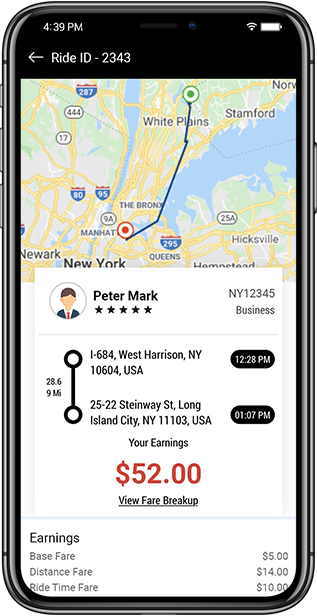A detailed screenshot captures a traditional style iPhone with a sleek, shiny black frame. At the top of the screen, against a black banner, white text reads "4:39 PM" in the left-hand corner. Adjacent to it are icons representing a Wi-Fi signal and a battery indicator. Below this banner, the display shows an arrow pointing left, and the text "Ride - ID: 2343."

The middle section of the screen features a map highlighting various locations including White Plains, Stamford, Newark, and Hampstead, as well as smaller towns, indicating a trip from one point to another. A white square on the map details information about a business called "Peter Mark," rated five stars. Accompanying it is a small person icon and text that reads "NY12345 Business," followed by the address "6484 West Harrison, New York, 10604 USA." The timestamp on this section reads "12:28 PM" with a distance of "28.69 miles."

Further down, another entry displays the address "25-22 Steinway Street, Long Island City, New York, 11103 New York" marked with the time "1:07 PM." The earnings for this trip are prominently displayed in red text as "$52." An option to "View Fare Breakdown" is available, listing the components of the fare: base fare, distance fare, and ride time fare.